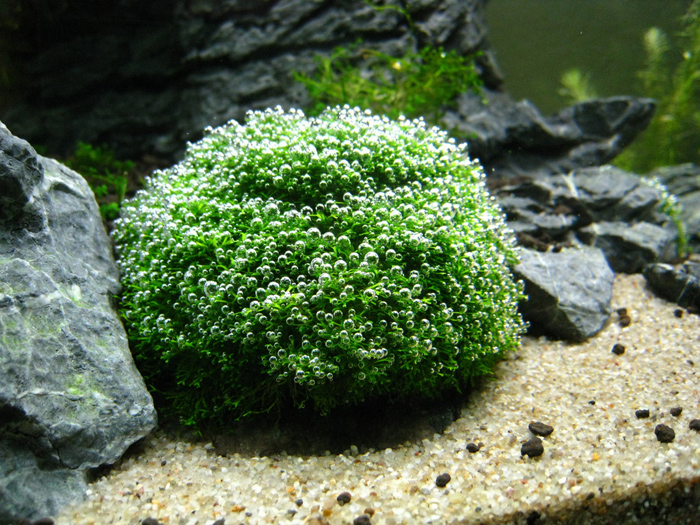The photograph captures an underwater scene, likely within an aquarium, where the main focal point is a green plant or algae-type organism adorned with numerous bubble-like circles. The base of the image is lined with light brown, orange, and white pebbles that cover the flat surface. Flanking the green plant on both sides and extending behind it are larger charcoal-gray rocks with sharp, angular edges. These rocks form a striking outcropping that rises in the background and is partially covered by additional green growth. The surrounding scene includes other weed-like plants, adding to the aquatic ambiance and depth of the setting.